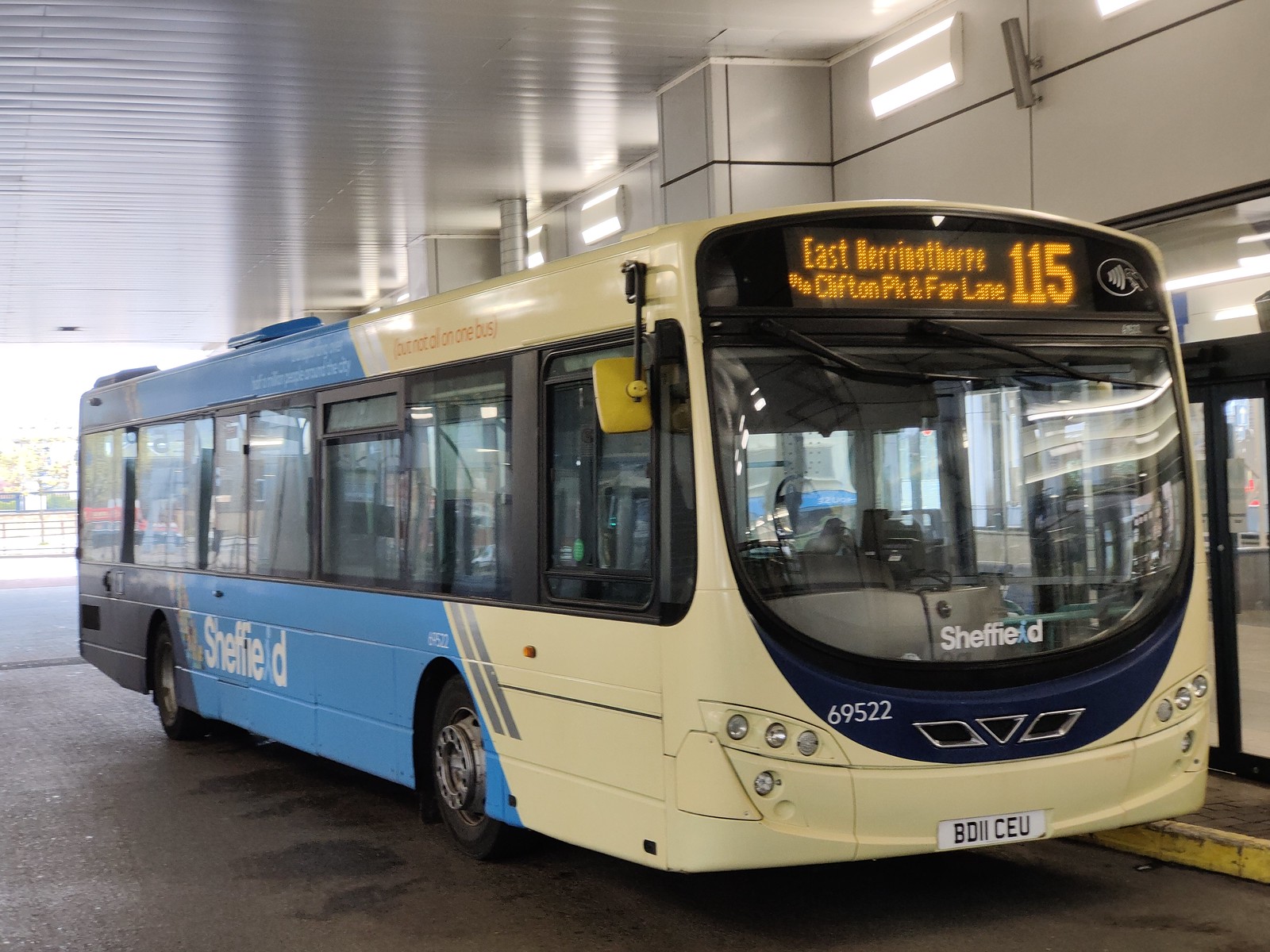This image features a city transit bus stationed under an awning at what appears to be a bus stop or station. The bus boasts a distinctive color scheme: the front section is light yellow, transitioning to blue towards the back, with a black rear. Prominently displayed above the windshield is an electronic sign that reads "East Herringthorpe via Clifton Park and Far Lane 115," indicating its route. Additionally, the front of the bus bears the name "Sheffield." The license plate is BD11CEU, and the bus number is 69522. Noticeably, the front of the bus is equipped with three small round headlights and two round blinkers, and its reflective windows suggest it is parked alongside a sidewalk.